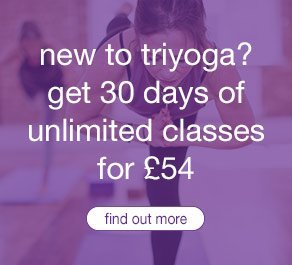The image is a square photo set in a yoga studio with a light-colored floor and features two women practicing yoga. The background shows a peaceful studio environment with a yoga mat in the foreground and another in the back left. Both women, who appear to be possibly Asian, are depicted standing on their left legs with their right legs extended behind them, leaning forward in a balanced pose. The woman in the foreground has dark hair parted in the middle, her hands clasped in front of her as she looks down in concentration.

A translucent purple overlay is applied to the image, giving it a serene and cohesive look. White lowercase text is centered prominently over the purple layer, reading: "new to TriYoga? get 30 days of unlimited classes for £54." Below this text, there is a white oblong button with the words "find out more" written in purple or blue, inviting viewers to learn more about the offer.